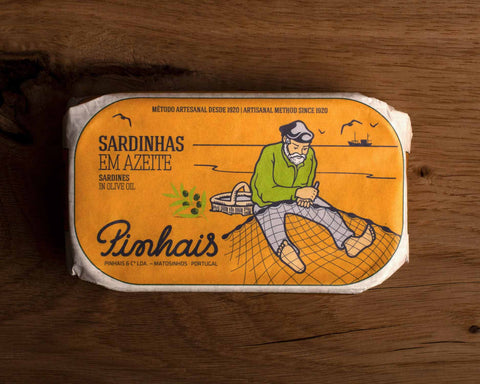This image captures a rectangular tin of sardines placed on a wooden surface, possibly a table or cutting board. The vibrant orange foil label on the tin features a detailed illustration of a fisherman. The fisherman, depicted with a gray beard and wearing a hat, lime green shirt, and gray pants, sits barefoot with his legs outstretched. He is focused on repairing a sardine fishing net that lies across his lap, using tools he holds in his hands. Behind him sits a small basket, possibly containing sardines or his tools. In the background, a fishing boat is visible along with four seagulls in flight. An olive branch with olives is placed to the side. The label also prominently features the text "Sardinhas M. Azete" in the top left corner and "sardines in olive oil" underneath it. "Penhas" is written in black print at the bottom of the label.